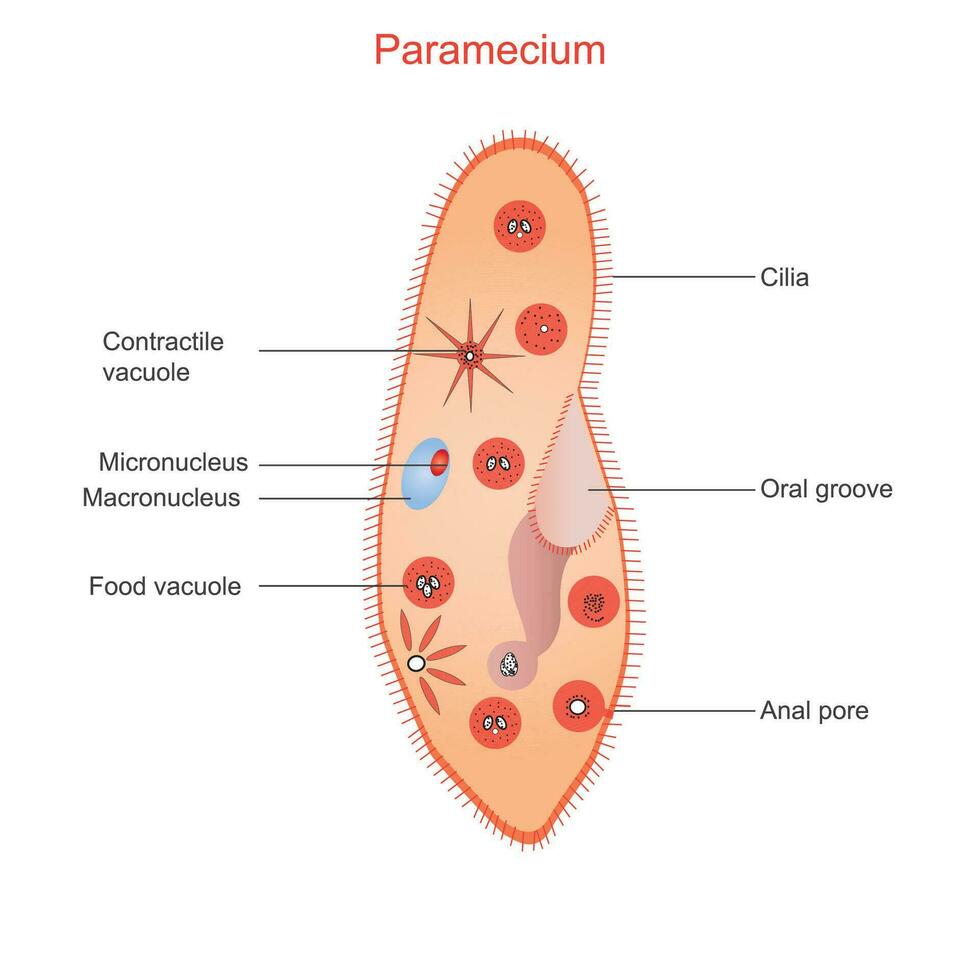This detailed medical illustration showcases a paramecium, prominently titled "Paramecium" in orange at the top. The organism is depicted vertically with an oblong, almost peanut-like shape, outlined in red. The interior is colored in shades of pink and beige, giving a somewhat organic appearance that might be reminiscent of skin or blood.

The outer edge of the paramecium is adorned with numerous hair-like structures known as cilia. Various internal structures are clearly visible and labeled in black text. These include the contractile vacuole, food vacuole, micronucleus, macronucleus, anal pore, oral groove, and cilia. Additionally, the diagram features smaller internal components like starburst shapes and blue blobs, providing a detailed cross-sectional view of the paramecium's anatomy.